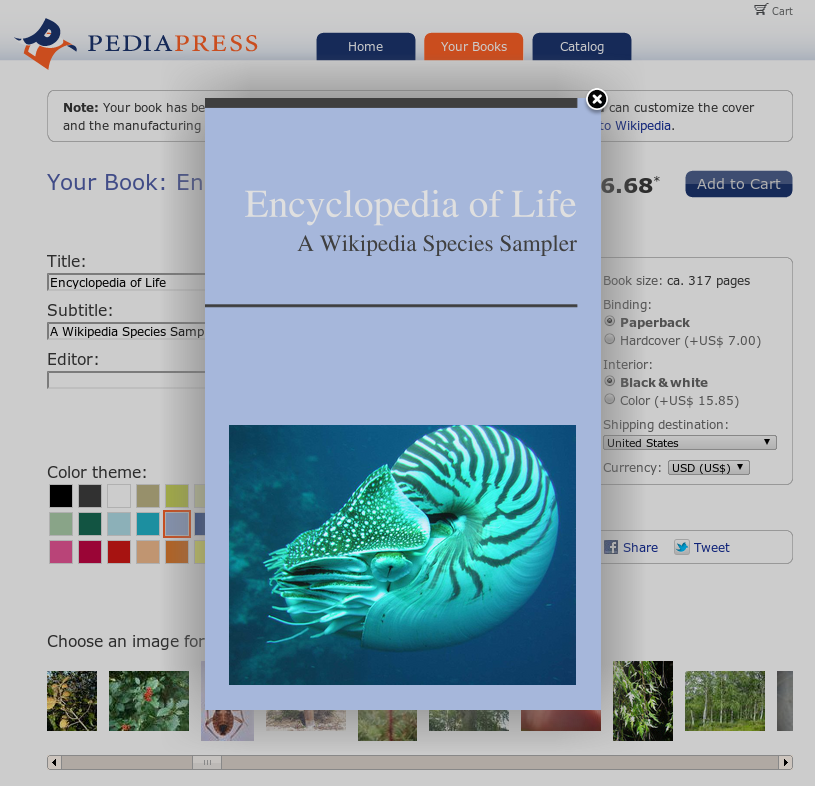The image depicts a webpage from PediaPress, an online platform for creating custom books. At the top of the page, "Pedia" is highlighted in blue while "Press" is in orange, alongside a matching blue and orange logo. The navigation bar includes three tabs: "Home" and "Catalog" in blue, and "Your Books" in orange.

Dominating the page is a prominent advertisement with the title "Encyclopedia of Life" in white text, promoting a "Wikipedia Species Sampler" in black text. Below the text is an image of a large sea snail or sea slug with a white shell marked by black lines and small protrusions.

This specific page allows users to purchase the "Encyclopedia of Life." It is available in paperback for $6.68 and in hardcover for $7.00. The book comprises 317 pages. Users can customize the book cover by selecting different themes and images provided on the page. This feature highlights the modern capability of personalizing printed content.